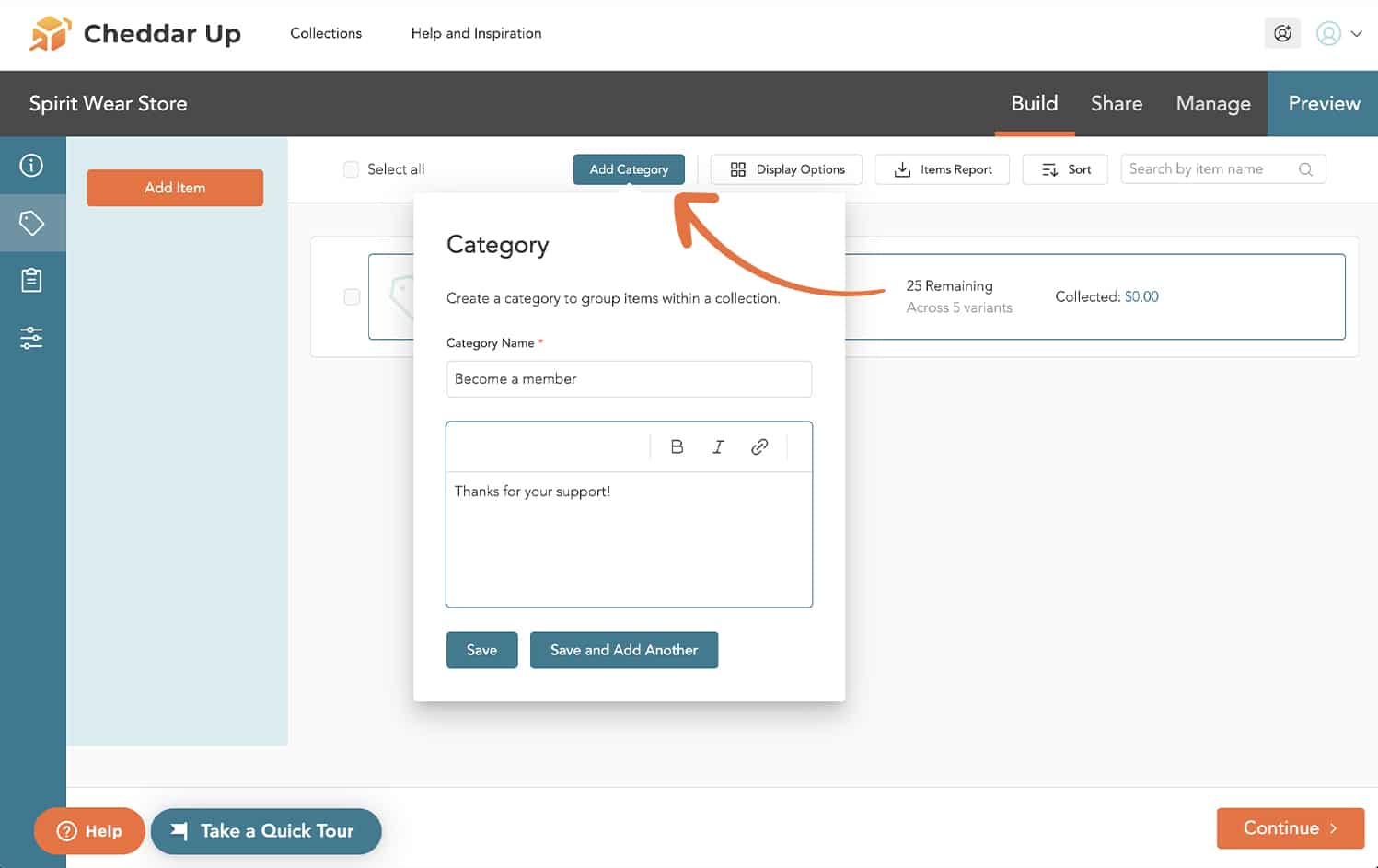The image portrays a webpage interface of the "Cheddar Up" platform, identifiable by its logo positioned at the upper left corner, which appears to be a stylized image of a pen or knife piercing a cube or block of cheese. The header reads "Cheddar Up Collections, Help and Inspiration". In the top right corner, there’s a profile or settings icon, accompanied by a drop-down menu featuring options for "Build," "Share," "Manage," "Preview".

Just below, additional menu items include "Add Category," "Display Options," "Items," "Report," "Sort," and a search function labeled "Search by Item Name". Dominating the center of the screen is a box highlighted with "Category" text, prompting users to create a category for grouping items within a collection. The box fields read "Category Name," with introductory titles such as "Become a Member" and "Thanks for your support."

On the left-hand side are links and options related to "Spiritware Store" and "Add Items," each represented with distinct icons for various actions. Towards the bottom of the interface, buttons such as "Continue," "Help," and "Take a Quick Tour" are available, guiding users through further steps and assistance options.